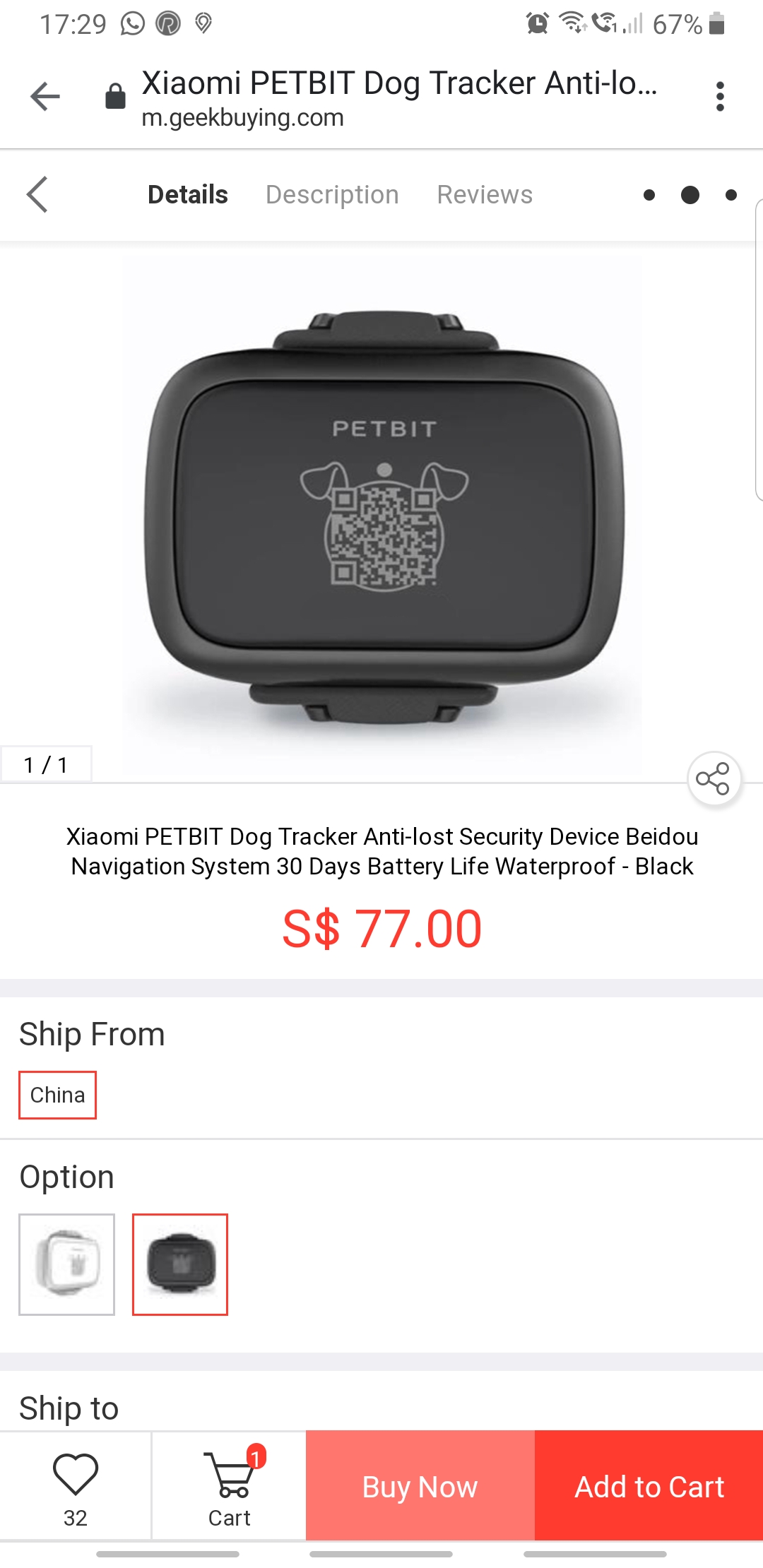A detailed screenshot of the m.geekbuying.com mobile website is displayed, showcasing a product listing for the Xiaomi PetBit Dog Tracker. The layout suggests it was captured on an Android device, evidenced by the icons for time (12:45), WhatsApp, clock, WiFi signal, cellular strength, and a battery status indicating 67% at the top of the screen. The web page features a clean white background, centrally displaying a single image of the dog tracker, which appears to be designed as a collar or bracelet.

The product, labeled Xiaomi PetBit Dog Tracker, is priced at 77 Chinese Yuan and is available in two color options: white and black. The item ships from China and has garnered 32 hearts, indicating interest or likes from users. In the lower portion of the screenshot, four icons are visible: a heart symbol with the number 32, a shopping cart symbol indicating 1 item in the cart, a pink "Buy Now" button, and a red "Add to Cart" button. It is not specified whether the item in the cart is the dog tracker being viewed.